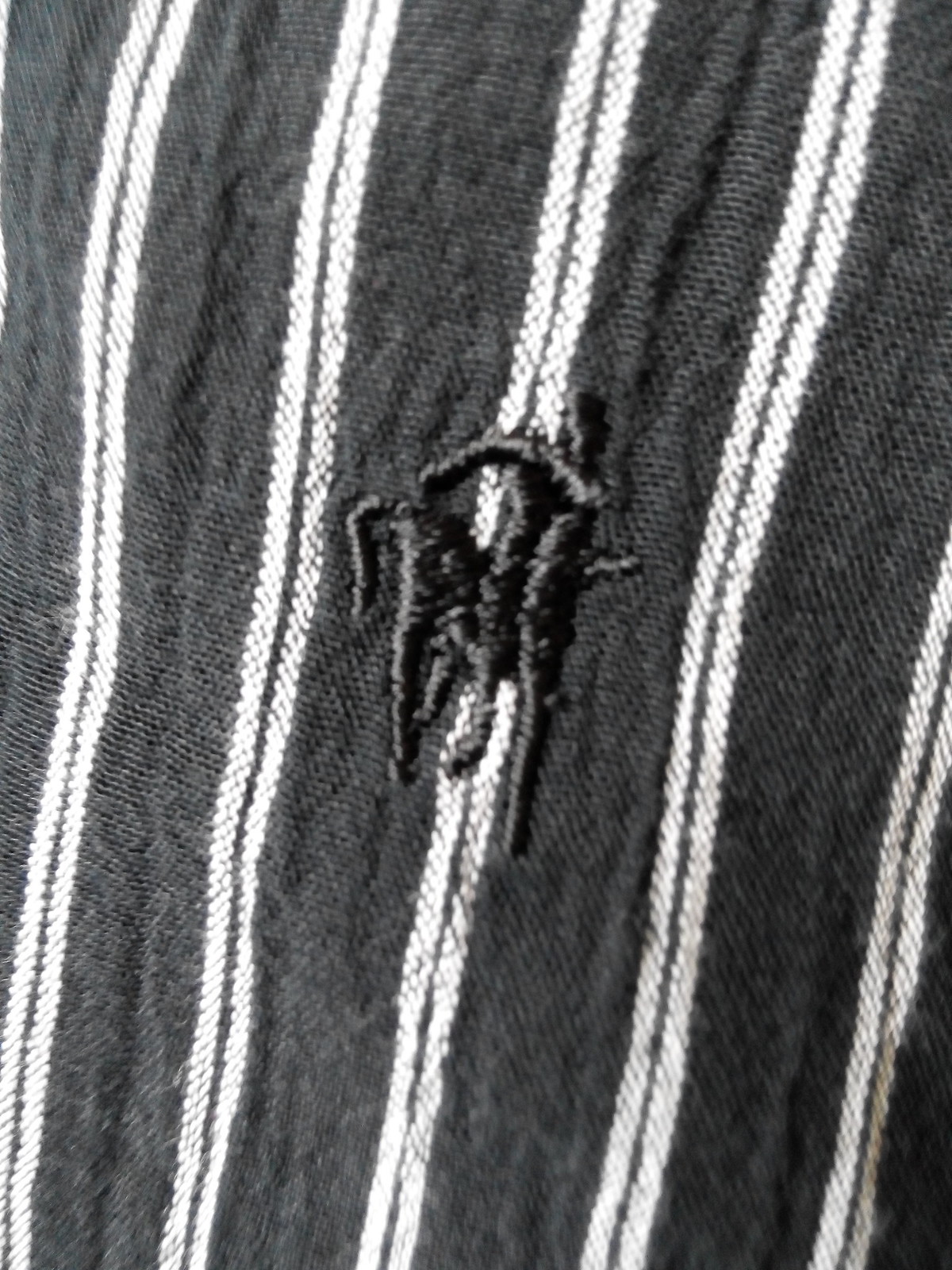This is a vertically oriented rectangular image showcasing a piece of fabric, likely clothing or a blanket. The fabric features a pattern of vertical stripes that run at a slight diagonal, angling from the bottom left to the top right. The prominent stripes are thick and gray, while in between them are very thin white stripes. Additionally, a thin gray line runs between each pair of white stripes. Embroidered onto the fabric is a black emblem portraying a person sitting on a horse, rendered in dark thread.